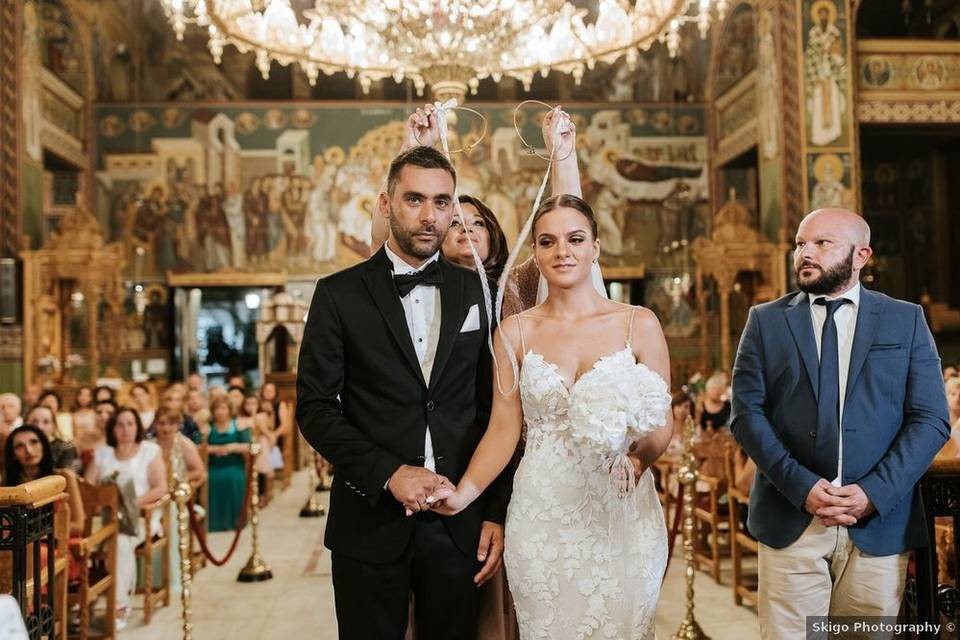In this vibrant wedding photograph, taken by Scego Photography, the main focus is the bride and groom standing hand-in-hand at the center. The groom, dressed in a black tuxedo with a white handkerchief in his pocket, gazes directly into the camera. The bride, in a white lace wedding dress and holding a white bouquet, looks off slightly to the left. Behind them, a woman holds up two hoops adorned with white ribbons, resembling halos over the couple’s heads. To the right of the couple, a man in a blue jacket, matching tie, and beige pants watches them intently. The scene is set in a grand, possibly church-like building, featuring an elaborate chandelier above and a mosaic on the upper balcony in the blurred background. Rows of spectators fill the space, witnessing the joyous occasion.